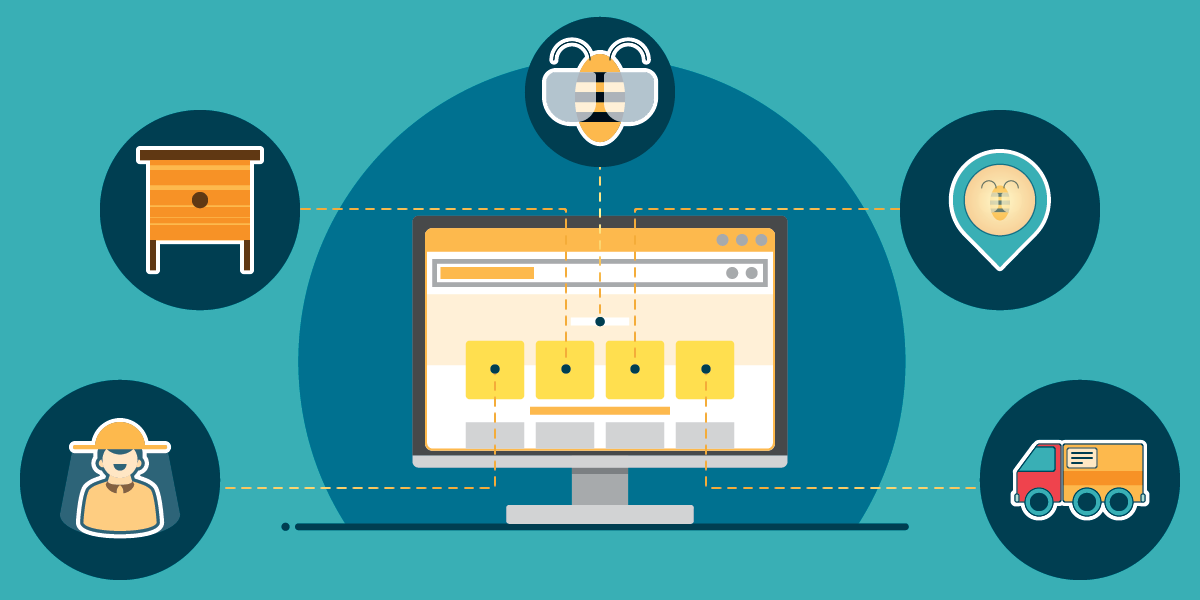In this digitally generated image, the backdrop features a light blue, aqua tone. Central to the composition is a horizontally rectangular section dominated by a darker blue, nearly complete circle. Positioned within this circle is a computer monitor which stands on a gray base and has a black frame. The monitor screen displays a series of yellow squares and suggests a loading bar.

Radiating from this central monitor are five dotted lines that extend outward to connect with five smaller dark blue circles. Each circle contains specific icons that collectively narrate a logistics network, possibly depicting the journey of honey from a hive to its delivery. In the top central circle, a yellow honeybee is illustrated. The upper-right circle portrays an upside-down teardrop, resembling a location pin, with a face in it. The lower right circle features a delivery truck bearing a cardboard box in its cargo area. On the left side, in the lower circle, there's an image of a man wearing a wide-brim hat, indicative of a beekeeper. Lastly, the circle on the far left shows a single-drawer dresser, reminiscent of a wooden hive.

The entire scene is rendered in a cartoon style, creating a cohesive visual representation that emphasizes the interconnectedness of these various elements through the use of blue hues and linear connections.